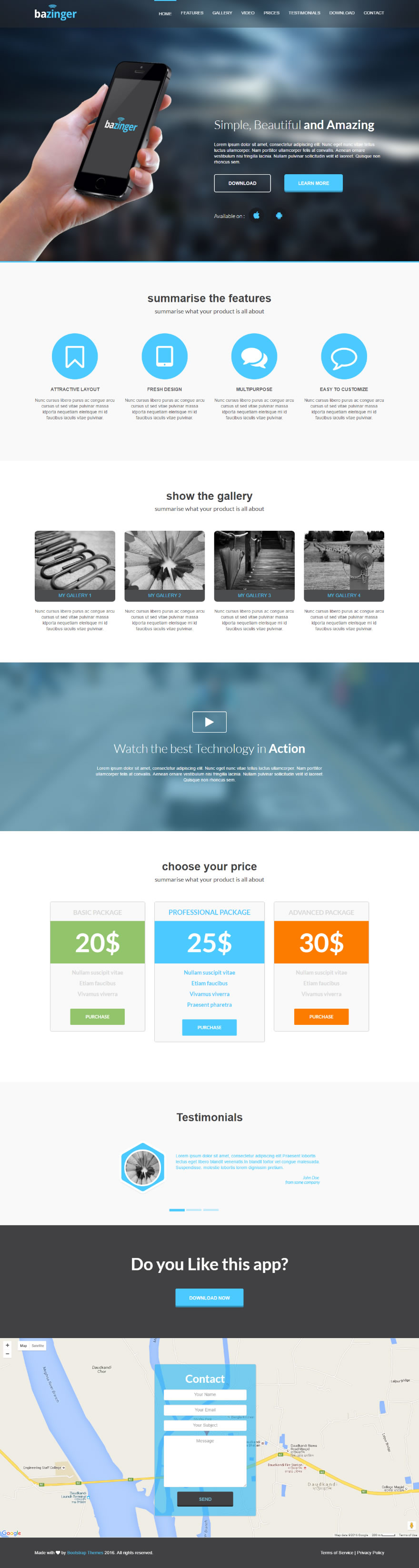A promotional image for Bazinger, a tech subscription service, is depicted in this photo. The Bazinger logo, prominently displayed at the top, features 'BA' in white and 'Zinger' in light blue font, all positioned towards the left side of the image. The screenshot is elongated, running from top to bottom. The tagline "Simple, Beautiful, Amazing" introduces Bazinger's main benefits, emphasizing its attractive layout, multipurpose functionality, and customization options.

The screenshot further highlights a gallery section, showcasing different pricing tiers: $20 with a green and white theme, $25 with a light blue and white theme, and $30 with an orange and white theme. Additionally, there's a call-to-action, inquiring if viewers like the app, and a contact option.

Towards the bottom, there appears to be a map, suggesting that Bazinger may include tracking features. A hand is holding a phone, implying practical, hands-on use of the application. The caption at the bottom reads, "Watch the Best Technology in Action," inviting users to view a video for more detailed information about the service.